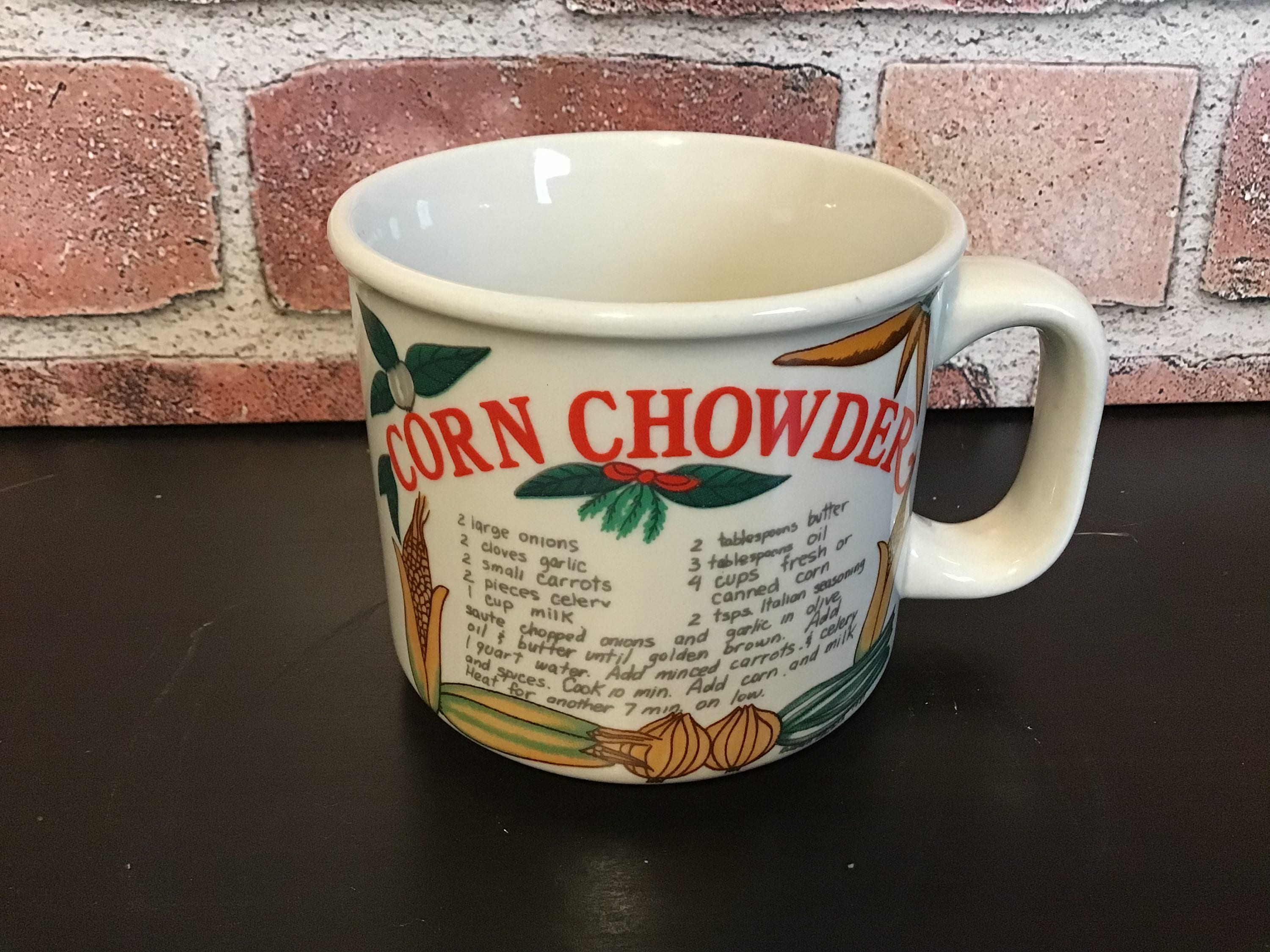The image features a close-up of a heavy, off-white ceramic mug, positioned on a dark brown, possibly black, countertop or floor. The background is dominated by a textured brick wall in light pinkish-red hues, with visible mortar lines. The mug prominently displays the words "Corn Chowder" in bold red lettering, surrounded by illustrations of various vegetables like onions, corn, carrots, and chilies. Below the illustrations, there is a detailed recipe for making corn chowder, listing ingredients such as three large onions, two cloves of garlic, two small carrots, two pieces of celery, a cup of milk, two tablespoons of butter, three tablespoons of oil, four cups of fresh or canned corn, and two teaspoons of Italian seasoning. The recipe also includes cooking instructions: sauté chopped onions and garlic in olive oil and butter until golden brown, add one quart of water, minced carrots, celery, and spices, cook for ten minutes, and then add corn and milk, heating for another seven minutes on low.